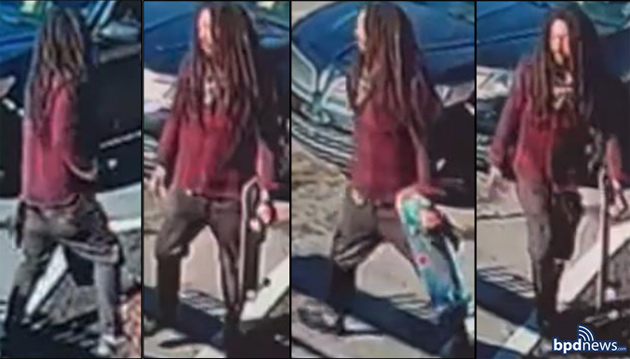The composite image from BPD News consists of four blurry security camera photos featuring a black man with long, blackish dreadlocks and a maroonish-red sweatshirt. The first panel on the far left shows him from behind, standing in front of a vehicle while wearing a brown jacket, black pants that sag below his rear end, and sneakers. The second panel captures him facing forward, holding a skateboard in his left hand, looking visibly angry. The third image shows him turned slightly, still holding the skateboard and appearing to walk towards someone, maintaining the angry expression. In the final panel on the far right, he is riding the skateboard, continuing to display the same angry demeanor. The images suggest a possible police search for this individual, potentially linked to an incident involving the skateboard.